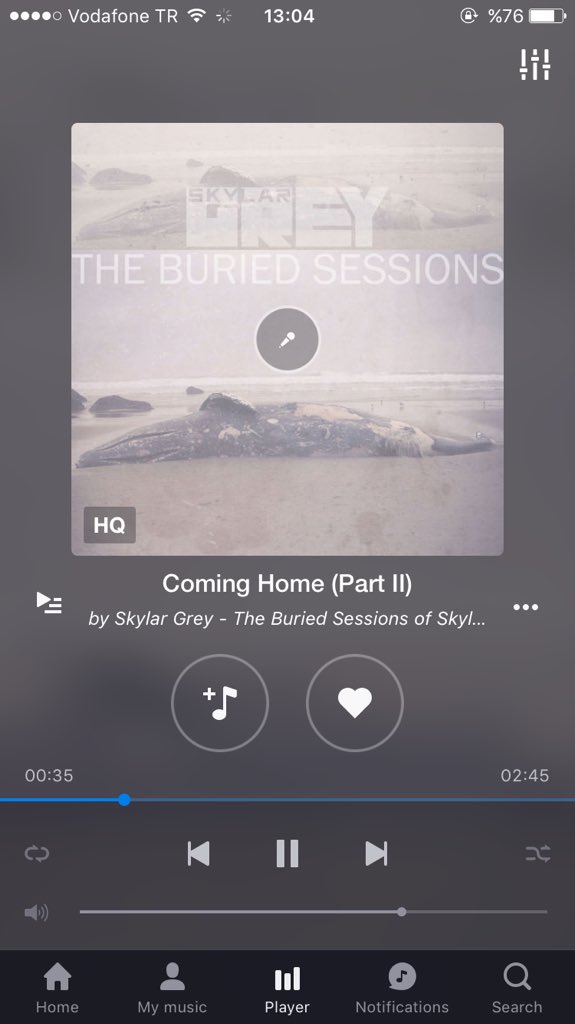The image showcases a mobile phone screen displaying a website. The phone indicates a battery level of 76% and the time as 13:04, with Vodafone as the network provider. The background is dark gray. At the top of the screen, there is a square image of a beached whale that has passed away, partially covered by sand. The text within the image reads "Dre, The Buried Sessions," and includes an "HQ" label. Below the image, it states "Coming Home Part Two by Skyler Gray, The Buried Sessions of Skyler." There are icons featuring a heart within a circle and a music note within another circle. The song has been played for 35 seconds out of its total duration of 2 minutes and 45 seconds, with options to pause, rewind, and fast forward. At the bottom of the screen, navigation options include Home, My Music, Player, Notifications, and a clickable search bar, with only one song displayed on this particular view.